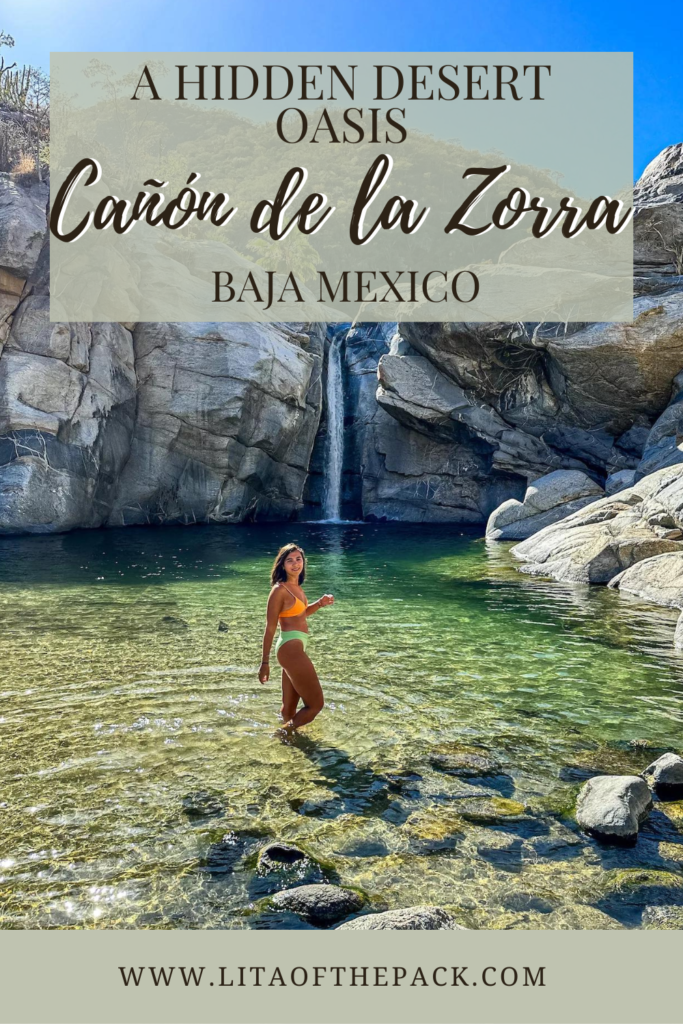A promotional poster showcases a breathtaking natural destination, featuring a stunning photograph of a young tan woman standing in a clear, green-toned pond with submerged legs. She has medium-length brown hair and appears to be in her late teens to early twenties. The woman is wearing an orange bikini top and lime green bikini bottoms. Behind her, a natural waterfall cascades down, framed by large stone formations, adding to the serene beauty of the setting. The text "A Hidden Desert Oasis, Cañon de la Zorra, Baja Mexico" is displayed at the top of the image in black font, while a gray horizontal strip at the bottom of the poster bears the text "www.litaofthepack.com".